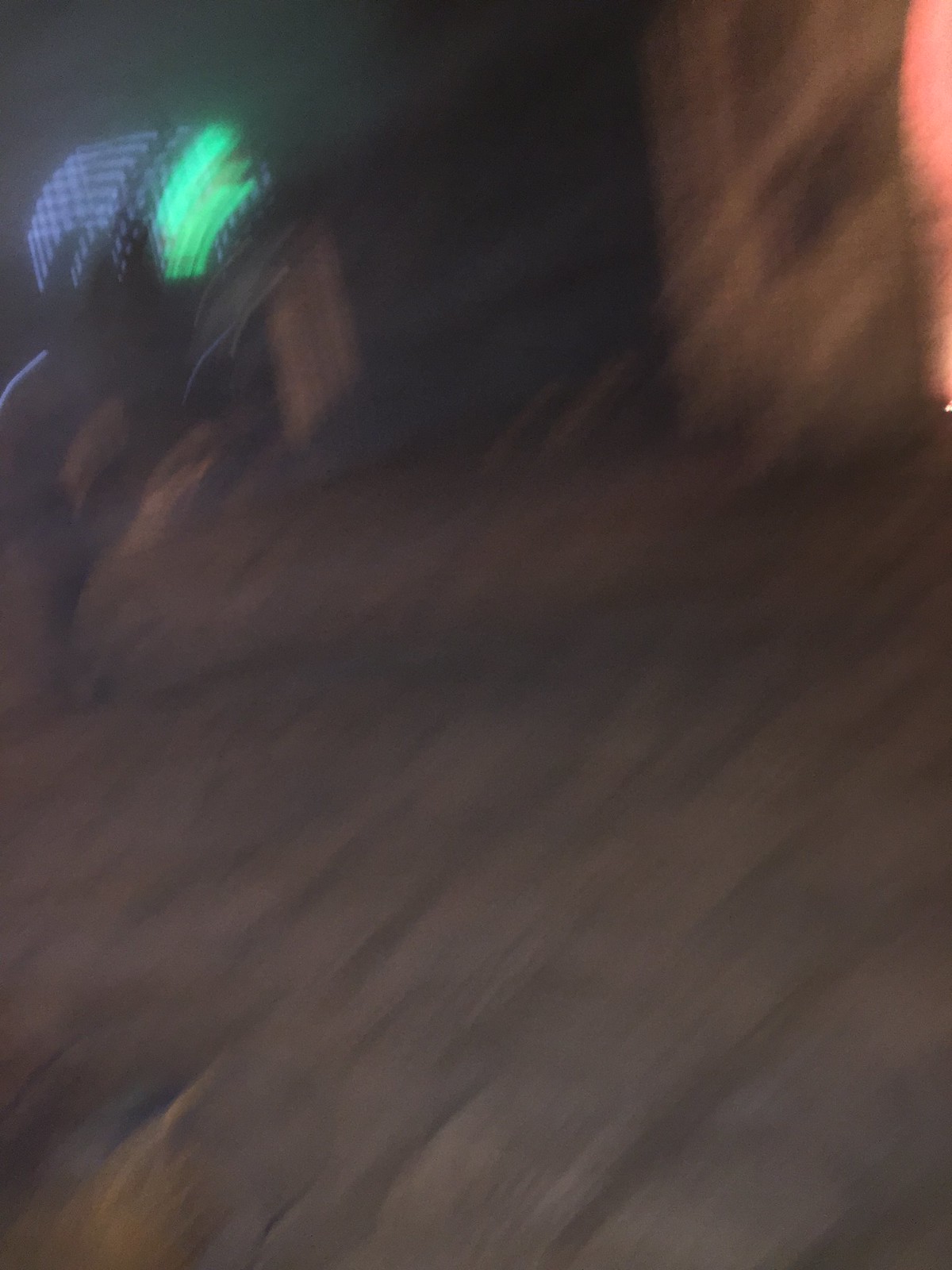The image is quite blurry, depicting what appears to be the floor of a room with a brownish-colored carpet. On the upper left-hand side of the image, an object with lights is partially visible. The top lights on this object shine in a purple hue, while the lights on the side emit a light green color. This object seems to have a wooden base. Along the upper right-hand edge, the corner of a wooden door is seen coming into the frame. To the right of this door, there is a pink-colored light, adding a touch of bright color to the scene.